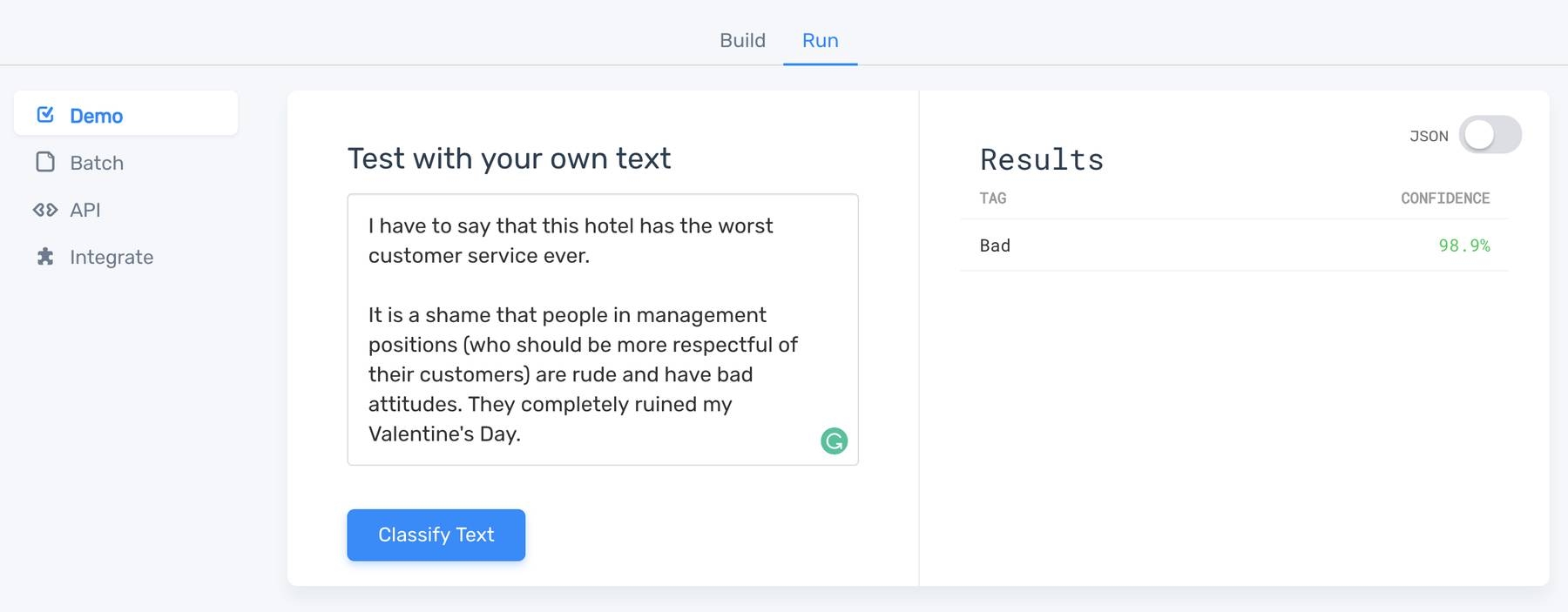**Screenshot of a Text Classification Demo Interface**

The screenshot showcases a portion of a webpage designed for a text classification demo. The interface prominently displays the phrase "Test with your own text" and contains several interactive elements. The user has navigated to the "Run" tab, one of the two available options alongside "Build." The screen also displays sections labeled "Batch," "API," and "Integrate," indicating different functionalities or steps in the process.

On the right side of the interface, a "Results" section is visible. Here, "350W" is displayed next to an on-off button, which is currently in the "off" position. Below this, a "Tag Confidence" rating shows a remarkably high confidence level of 98.9% for the classification of the text as "bad."

The user's input text criticizes the customer service of a hotel, stating, "This hotel has the worst customer service ever. It is a shame that people in management positions who should be more respectful of their customers are rude and have bad attitudes. They completely ruined my Valentine's Day."

Additionally, the webpage appears to have the Grammarly extension installed, which suggests possible textual improvements.

Overall, the screenshot captures a detailed view of a text classification demo, highlighting user comments, interactive elements, and performance metrics.